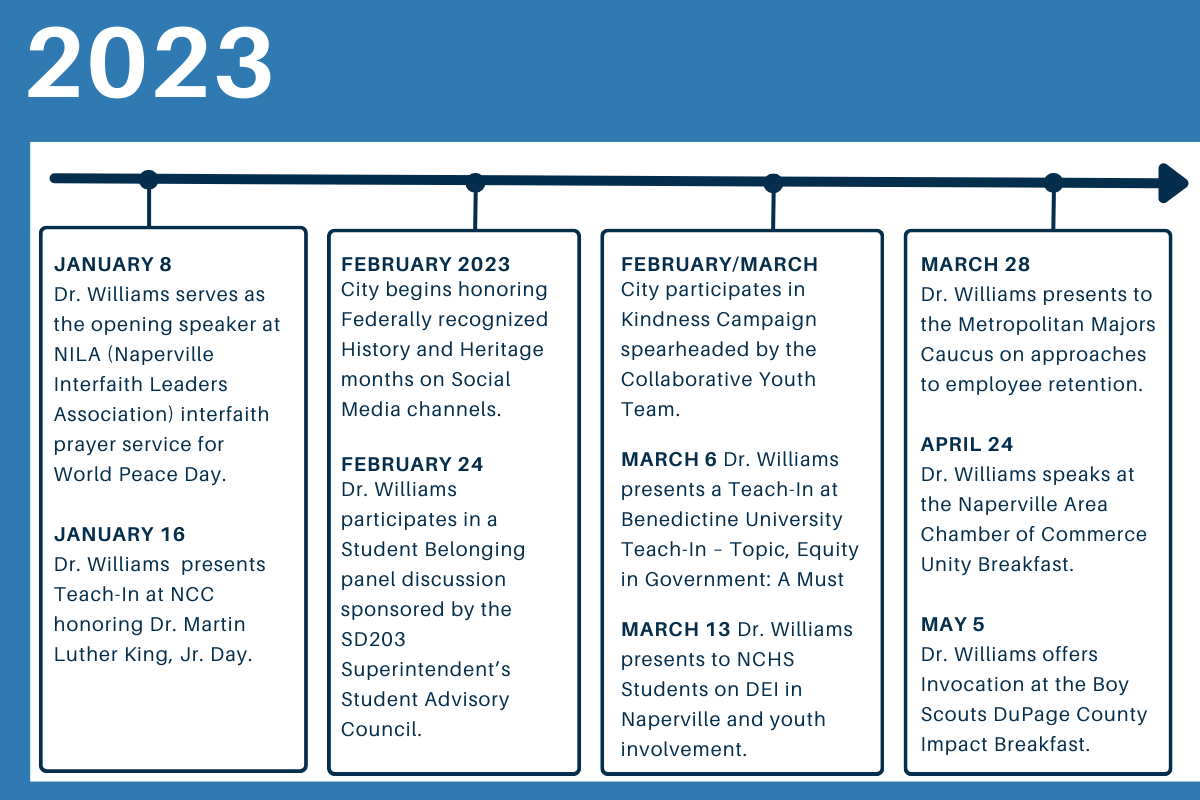The image is a detailed 2023 calendar or timeline of events featuring Dr. Williams, presented with a blue border that is thicker on the top and thinner on the sides and bottom. At the top left corner, "2023" is prominently displayed in white text. A black horizontal line with an arrow on the right runs across the image, below which are multiple bordered paragraphs connected by lines descending from small circles. The events are listed chronologically, starting from January 8th and continuing through to May 5th.

In the first section, dated January 8th, Dr. Williams serves as the opening speaker at the Naperville Interfaith Leaders Association (NILA) Interfaith Prayer Service for World Peace Day. January 16th notes that Dr. Williams presents a teaching session at North Central College, honoring Dr. Martin Luther King Jr. Day.

The second section covers February, indicating that Citi begins to recognize Federally Recognized History and Heritage Month on their social media channels. On February 24th, Dr. Williams participates in the Student Belonging Panel Discussion, sponsored by the SD203 Superintendent Student Advisory Council.

In the third panel, events continue in March with a significant date on March 6th and March 13th. March 28th is another notable event date, as is April 24th.

The timeline concludes with a final date of May 5th, where Dr. Williams offers the invocation at the Boy Scouts' DuPage County Impact Breakfast. The detailed itinerary highlights a series of engagements and contributions by Dr. Williams throughout the first half of 2023.